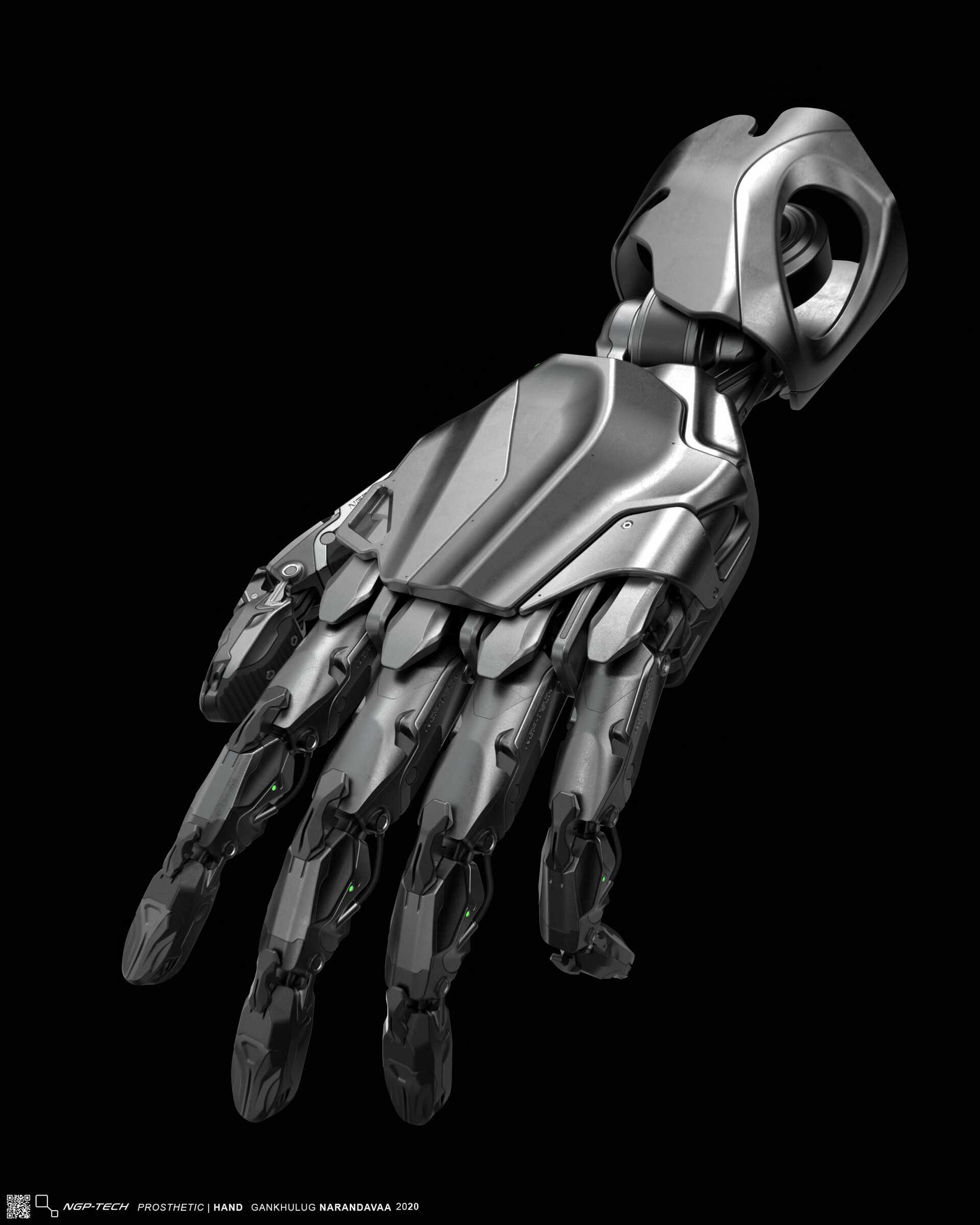The image showcases a highly detailed and realistic rendering of a silver, robotic prosthetic hand, designed with anatomical accuracy to replicate the structure of a human hand. The prosthetic features articulated fingers with multiple joints and segments, and an opposable thumb. The hand is composed of various shades of gray and silver metallic components, complemented by sleek black accents, lending it a modern and high-tech appearance. Each joint is intricately designed with small green lights, possibly indicating sensors or status indicators. The palm and the back of the hand are reinforced with robust, armor-like plating, enhancing its sense of durability. The wrist section transitions into a rounded compartment with an opening, designed for attachment to a human arm. The background is a solid black, which highlights the hand’s intricate details and illumination. The bottom left corner of the image contains text that reads "NGP Tech Prosthetic Hand Genkulag Narada 2020," along with a QR code and a graphic of two squares connected by a slanted line. The overall composition is rectangular in shape, presenting a futuristic and technologically advanced prosthetic hand.